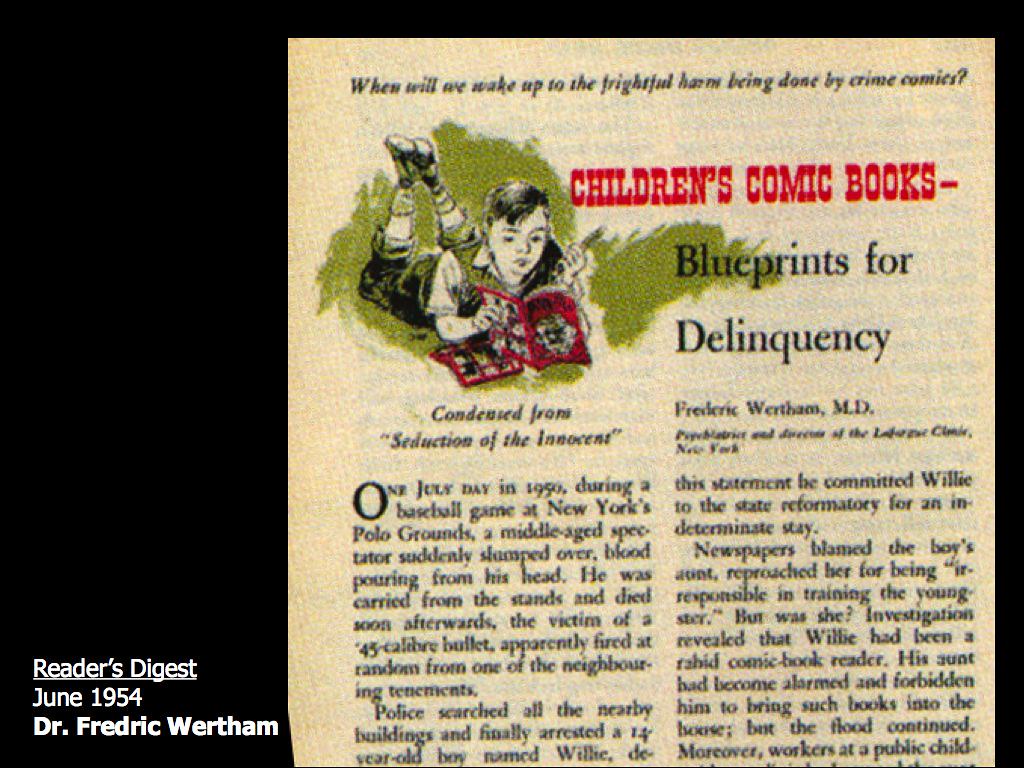This image features a digitized version of a vintage Reader's Digest article from June 1954 by Dr. Frederick Wertham, displayed on a black background. The lower left corner of the image is marked with white text indicating "Reader's Digest, June 1954, Dr. Frederick Wertham." The main article page, a tan-colored paper, prominently showcases its title in black at the top: "When Will We Wake Up? To the Frightening Harm Being Done by Crime Comics." Below this title, an illustration depicts a young boy lying on his stomach with his feet up, reading a red comic book with a flashlight. In bold red and black text, the header reads, “Children’s Comic Books: Blueprints for Delinquency,” suggesting the article's critical stance on the negative influence of crime comics on children. The article, condensed from Wertham's "Seduction of the Innocent," starts with a story underscoring the potential for juvenile delinquency influenced by comic books, highlighting an incident involving a boy named Willie in New York. The remaining content continues in columns, critiquing the alleged corrupting nature of comic books on young readers.